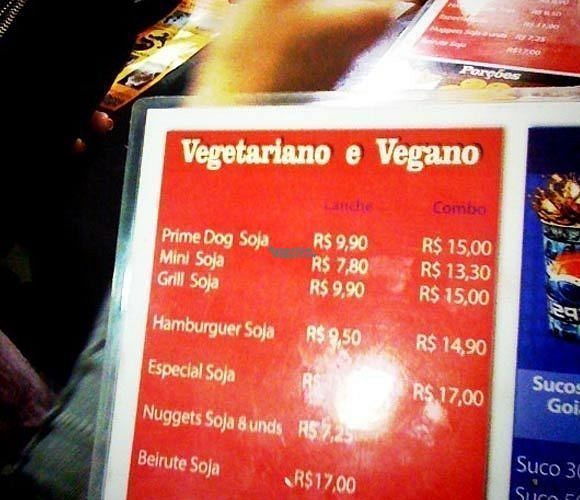The image depicts a laminated menu with a distinct white border. The left portion of the menu has a red background with bold white text and lists various vegetarian and vegan items under the heading "Vegetariano y Vegano." The right side of the menu has a blue background that appears largely cut off, but part of a Pepsi logo can be seen. 

On the red side, items are vertically listed: "Prime Dog Soja," "Mini Soja," "Grilled Soja," "Hamburger Soja," "Especial Soja," "Nuggets Soja," "8 Unds," and "Bayruta Soja." Each item has two prices: one for the standard serving and another for a combo. For instance, "Prime Dog Soja" is priced at R$9.90 standard and R$15.00 for a combo. Other prices include "Mini Soja" at R$7.80 and R$13.30, "Grilled Soja" at R$9.90 and R$15.00, and "Hamburger Soja" at R$9.50 and R$14.90. "Especial Soja" and "Bayruta Soja" combos are priced at R$17.00, though "Especial Soja" has a glare that obscures its standard price. "Nuggets Soja" at 8 units (8 Unds) costs R$7.25, with no combo price listed.

The blue side of the menu likely lists beverages, as inferred from part of the visible Pepsi glass with a cola splash, though the text is mostly unreadable due to it being cut off on the right. The background behind the menu includes a black area, a blurred hand, and possibly another menu or object adding to the visual context.